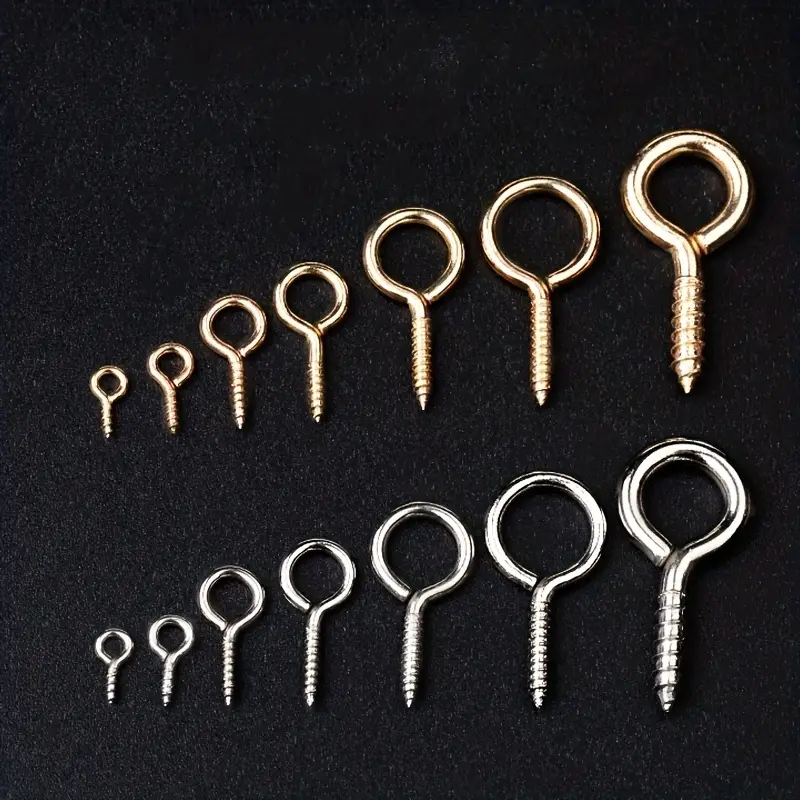The image depicts a color photograph of two parallel rows of screws meticulously laid out on a black surface. Each row consists of screws arranged from smallest to largest, with a total of seven different sizes per row. The top row features brass screws, while the bottom row showcases identical screws in a silver hue, either steel or another metal. Each screw is characterized by a circular or ring-shaped top, which differentiates them from typical screw heads and suggests they could be tightened by hand or with a tool. The screws appear new and unused, with various types of threads that differ based on size—the largest screws have threads set farther apart compared to the smaller ones. The overall aesthetic and precise arrangement highlight the distinct colors and sizes of the screws, creating a visually engaging composition without any additional text or description.